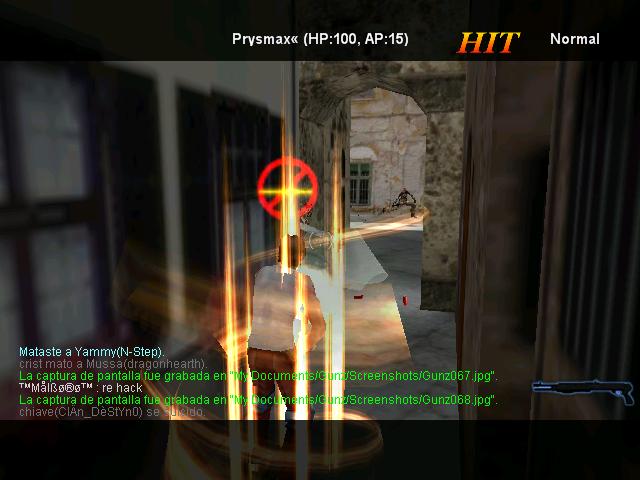The image is a blurry screenshot, likely taken of a video game displayed on a TV or computer screen. At the top, text indicates "Period Mac HP 100 AP 15 HIT Normal," suggesting gameplay details. The scene captures a stone walkway with an arched doorway, stone walls, and a window. There's a figure standing with their back to the camera, dressed in a white shirt and pants. Central to the image is a distinct red circle with a yellow cross. The bottom of the screenshot features green and blue text, likely file names, with a reference to a .JPG format. The background includes brown wooden elements and streaks of yellow light, which give the impression of a bronze or reflective surface. The image is partially obscured by vertical streaks of light and possibly glass or plexiglass elements, making some details difficult to discern accurately.